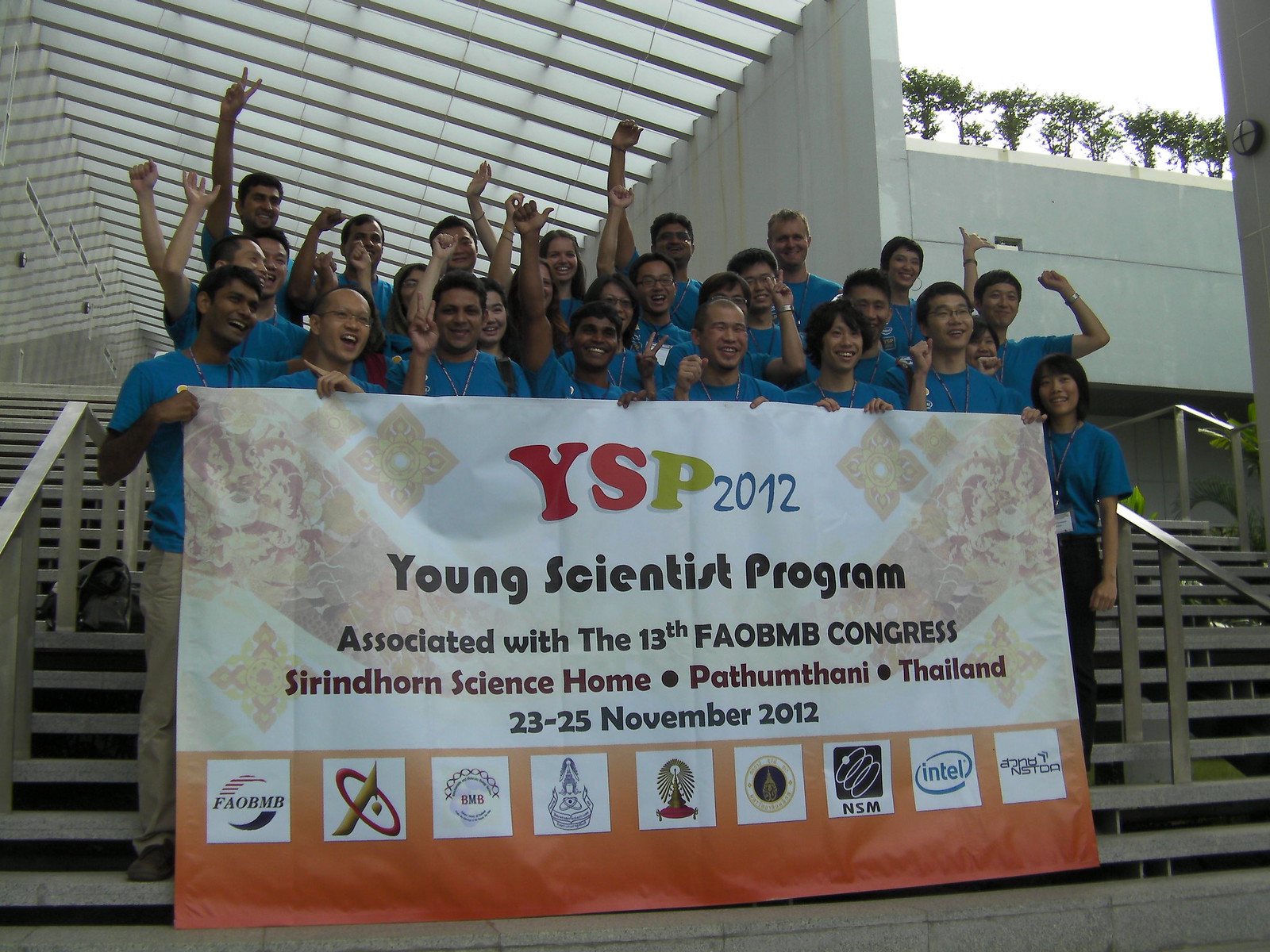A group of approximately twenty individuals, all of Asian descent—possibly Indian or Thai—are gathered on a grand staircase, each wearing a coordinated outfit consisting of blue shirts and lanyards. They stand proudly, holding a large banner that reads, "YSP 2012: Young Scientist Program, associated with the 13th FAO BMB Congress, Windhorn Science Home, Pathum Thani, Thailand, 23-25 November 2012." The background showcases the top levels of a substantial building, with the tops of trees visible beyond. Along the bottom of the banner, several company logos, including Intel, are prominently displayed, indicating sponsorship and support for the event. The overall scene exudes a sense of unity and scholarly purpose among the participants.